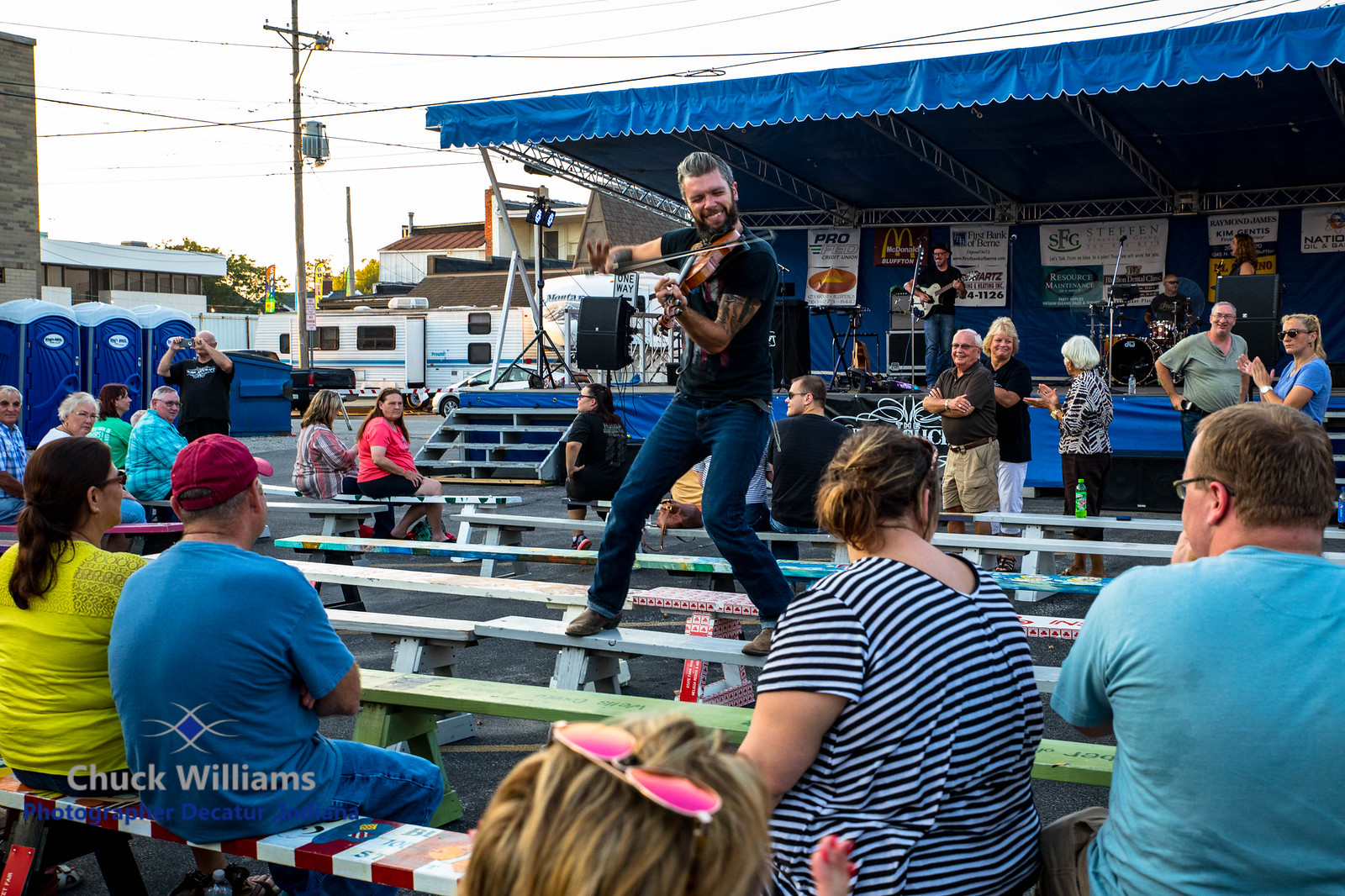In this vibrant outdoor photograph taken by Chuck Williams in Decatur, we see a lively crowd seated on several colorful benches with some green, red and white striped, and white benches. People are dressed in summer attire, enjoying the event. At the forefront, a charismatic figure with slicked-back hair and a black beard stands prominently on a white bench, playing a violin. His bow is in his right hand, resting on his left shoulder, and he’s dressed in a black t-shirt showcasing tattoos on his left arm, paired with blue jeans and brown shoes. He is smiling and captivating the audience’s attention. Behind him, a large stage under a blue canopy hosts several musicians, including one holding a white guitar. The background also reveals trailers and several port-a-potties beneath a hazy white sky. To the left, some buildings are visible, enhancing the setting's depth and context. The photograph is marked with "Chuck Williams Photographer Decatur" at the bottom left corner.